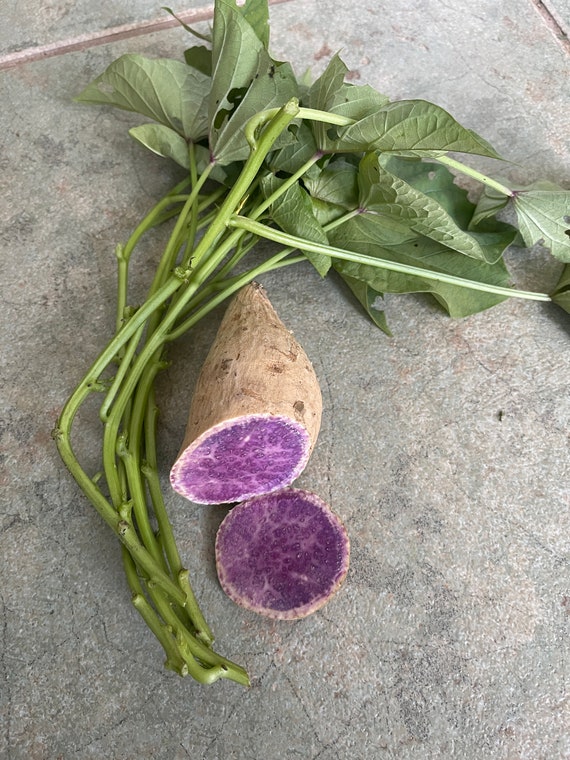The image depicts a stalk of what appears to be spinach laying next to a beet that has been cut open on a gray, cracked concrete floor. The beet has a light tan exterior with a vibrant purple interior, and a slice with the purple core facing the camera. Nearby, the spinach leaves, which appear dry and slightly wilted, are starting to fold together and their stems look limp, suggesting they are not freshly cut. The concrete surface is mottled gray with small fractures and darker gray cracks, some grout visible in between the slabs. There is a notable black spot on the ground to the right of the beet. The spinach is positioned to the left of the beet, arching from the bottom left to the top right, and its leaves display prominent veins. The color contrast between the limp, vibrant green stems and the duller green leaves further enhances the details in the image.